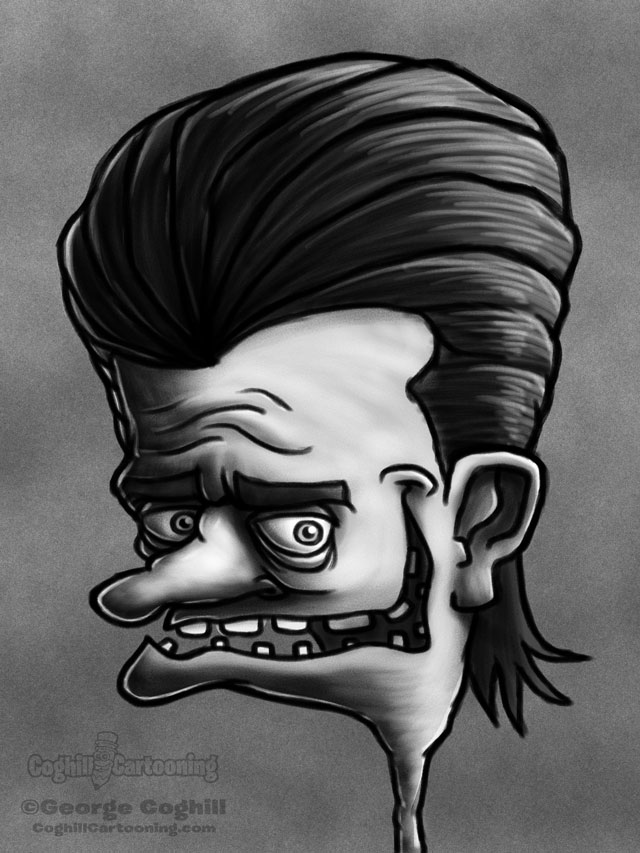Illustrated in an exaggerated, cartoonish style, this black-and-white image showcases a man's large, q-tip-shaped head with a significantly skinny, narrow neck. The man is facing left but directs his half-lidded gaze straight at the viewer, emphasizing his goofy facial expression. His slicked-back, black pompadour hair, accented with gray highlights, adds to his caricature-like appearance. Distinct forehead wrinkles and thick black outlines enhance the cartoony effect. His nose is notably long and pointy, contrasting with his wide, gapped smile that reveals spaced-out, white teeth. Set against a grainy, light gray background, the illustration captures a whimsical profile of this character. In the bottom left corner, there's a logo featuring a cartoon pencil accompanied by the text "Coghill Cartooning," followed by "Copyright George Coghill" and "coghillcartooning.com," all rendered in bubble letters.